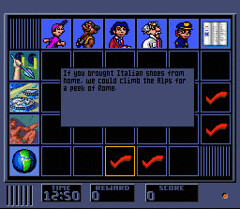This image is a grayscale screenshot from an unspecified video game. Central to its layout is a prominent gray text box with black script that reads, "If you brought Italian shoes from home, we could climb the Alps for a peak of Rome." Surrounding this text box is a grid of 35 smaller square boxes. Across the top row of this grid are six character images, each unique in appearance and attire: a fair-skinned individual in a white shirt and cap, a person with dark skin in a green vest, a possibly Latino character with chin-length curly hair in a red blazer and blue tie, a whimsical Einstein-like figure with wild hair, glasses, and a lab coat, a curly red-haired policeman with a blue hat and badge, and an icon suggesting a document or newspaper.

On the left side, descending vertically, are four images: a hand holding a spear, two coins on a yellow surface, a segment of Leonardo da Vinci's classic naked man painting, and an image of the Earth depicting blue oceans and green land. The bottom of the image displays several black boxes, including those labeled "Time 1250," "Reward 0," and "Score 0." Additionally, four of the boxes in the grid have red check marks in them—two on the right and two at the bottom—contributing to the game's visual indicators and overall interface.